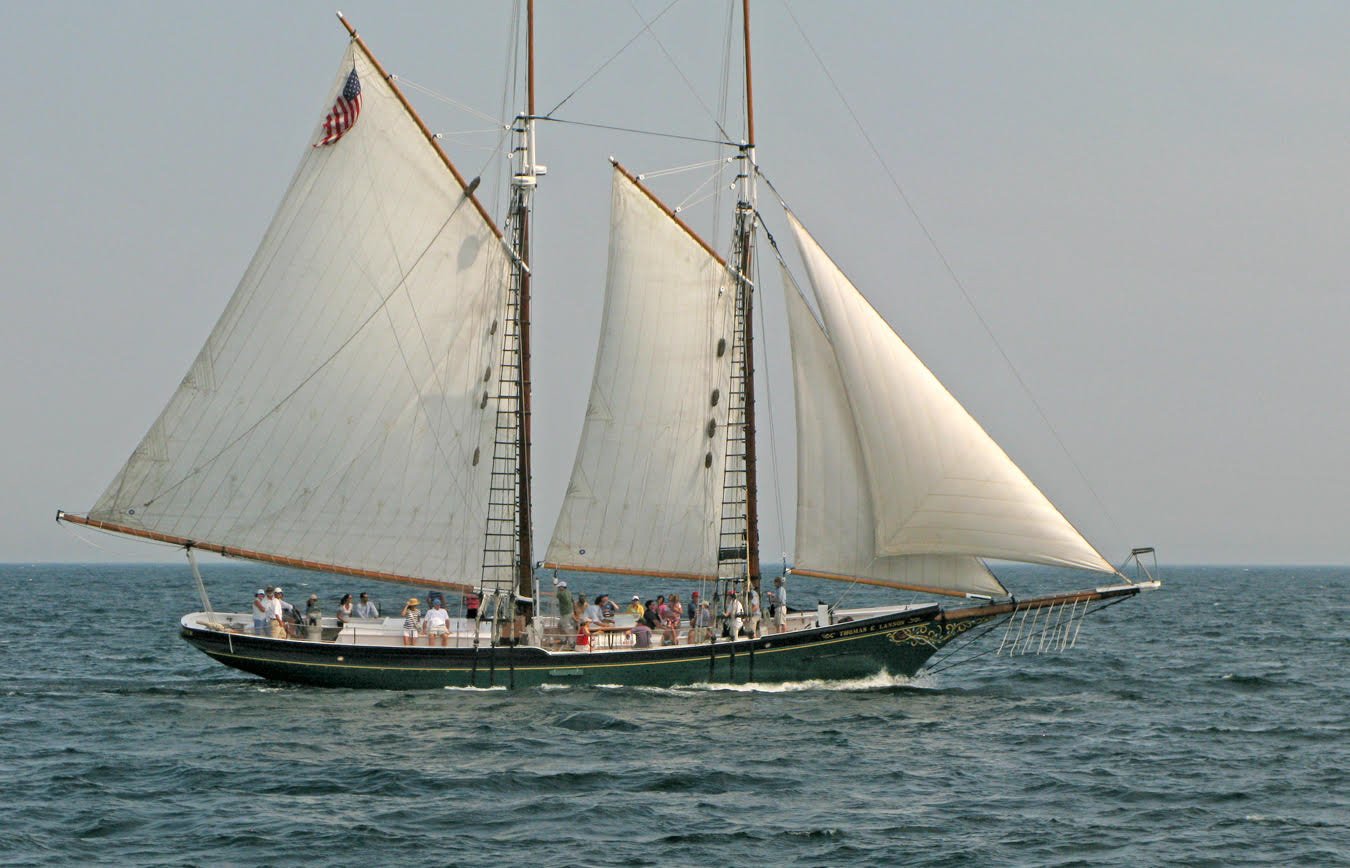The image captures a detailed and close-up view of a large sailing boat on vibrant greenish-teal ocean waters, set against a soft, grayish-blue sky devoid of clouds. The sailboat, front and center, is distinctly characterized by its dark green body adorned with a gold trim and topped in black, with a white interior. Notable is a sharp, long brown extension with a white tip protruding from the bow, where two of the four sails are fastened. The boat features four sails: two triangular ones facing forward on the front mast, with an additional one facing back, and a larger sail on the aft mast, topped with an American flag. The vessel is populated with around 15-20 individuals, though the distance makes their specific features indistinct. They stand in various vibrant outfits, including shirts and hats in shades of pink, yellow, and red, scattered across the boat. The scene exudes a lively yet serene maritime atmosphere, highlighted by the sailboat's elegance and the understated beauty of the open sea and sky.